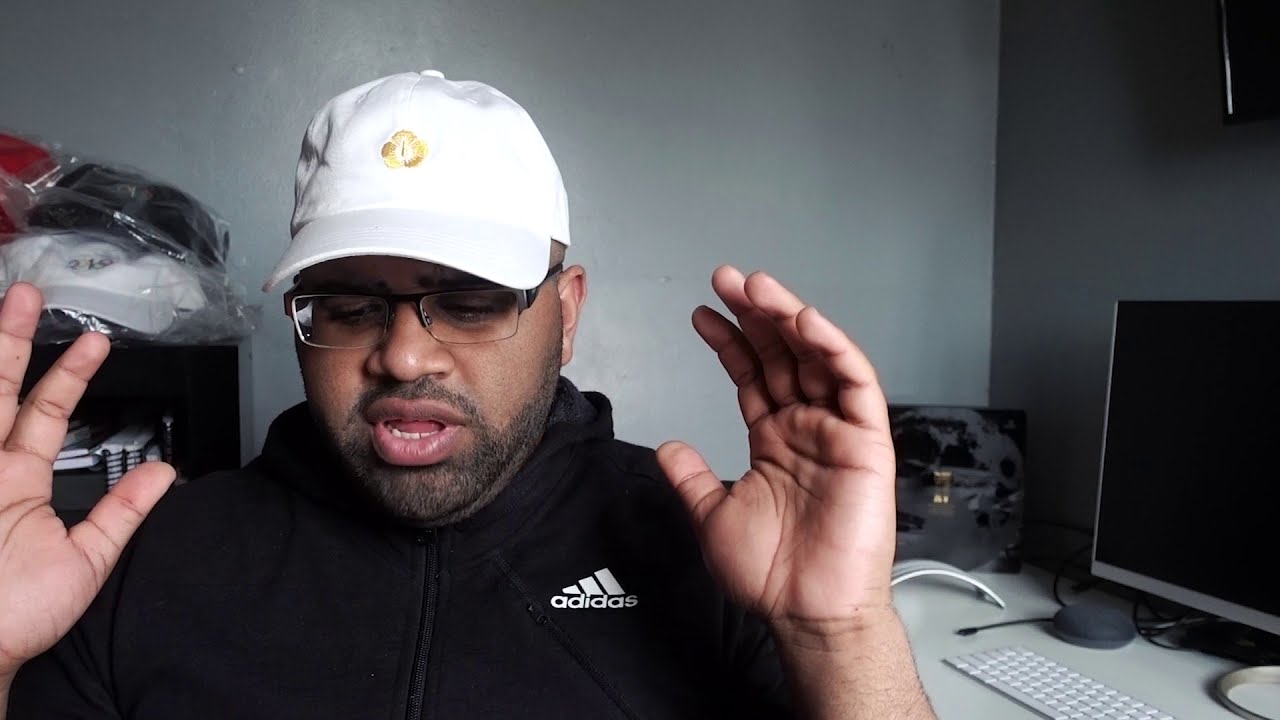The image features a dark-skinned man sitting on the left side, seen from the chest up. He is wearing a white baseball hat with a gold icon in the center and rectangular glasses. He has a short beard and is dressed in a black Adidas zip-up jacket with the logo and the word "Adidas" in white on the right side of his chest. His hands are raised towards his head in a gesture of disbelief or explanation, and his mouth is open as he looks down. To his right is a white Apple keyboard and a large monitor on a white desk. Behind him, the room has gray walls and a shelf on his left holding white, black, and red hats encased in plastic.